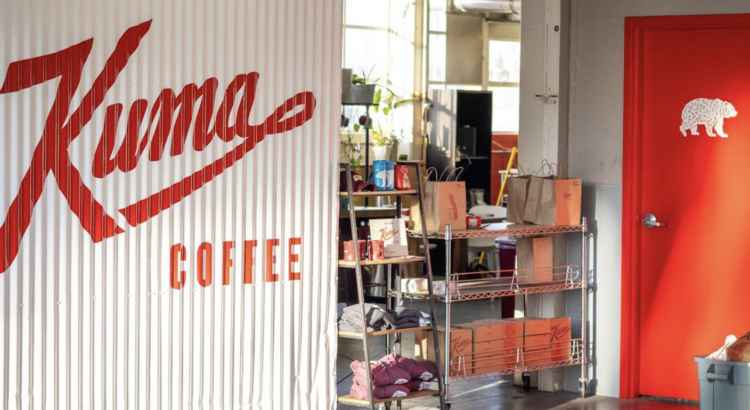The image depicts a coffee shop, specifically Kuma Coffee, as indicated by the large red lettering on a textured white wall made of corrugated metal on the left side of the image. Prominently positioned on the right side is a reddish-orange door with a white image of a bear, likely the company logo. The space also features several black shelving units, displaying a variety of merchandise including folded t-shirts, hoodies, mugs, and food packaging such as brown paper bags and cardboard boxes for takeout items. In the bottom right corner, there is a gray tub filled with various items, possibly a trash can. The overall setting suggests this might be a backroom or a staff area of the coffee shop, given the visible crates, shelving, and potential kitchen tools such as ladles in the background, indicating a functional space supporting the coffee shop's operations.